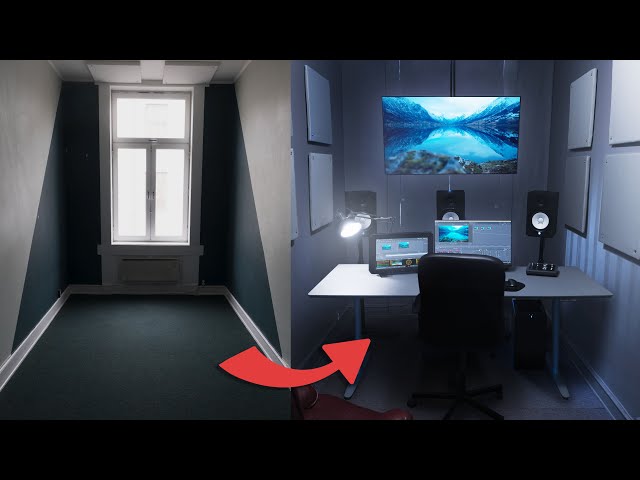This image portrays a detailed transformation of a small room with two distinct areas. On the left side of the image is a smaller room characterized by a large window with a top panel that is a wide rectangle and a lower panel comprising two tall rectangles. The walls of this smaller room feature a dark green paint that extends from the window and narrows into a triangular shape, transitioning into gray towards the front. The wall edges are adorned with white baseboards. The floor is dark, possibly black or very dark gray, and the ceiling is painted gray. A prominent red arrow is drawn from this room with the window, leading into a newly transformed office space on the right.

The office space highlights a steel desk with tubular legs, on which a large computer monitor and a smaller one are placed. To the left of the desk, a black office chair is visible from the back. Behind the desk stand three elevated speakers, and a desk light is positioned on the table. Mounted on the wall above is a large screen or monitor displaying an image of water and mountains. The walls of the office are medium gray, adorned with light gray sound squares. The entire transformation is emphasized by the juxtaposition of the previously empty, green-walled room with the fully equipped, modern office space.

This detailed caption synthesizes the shared and prominent features described across the three provided captions, highlighting the contrast and transformation of the room to an office space.